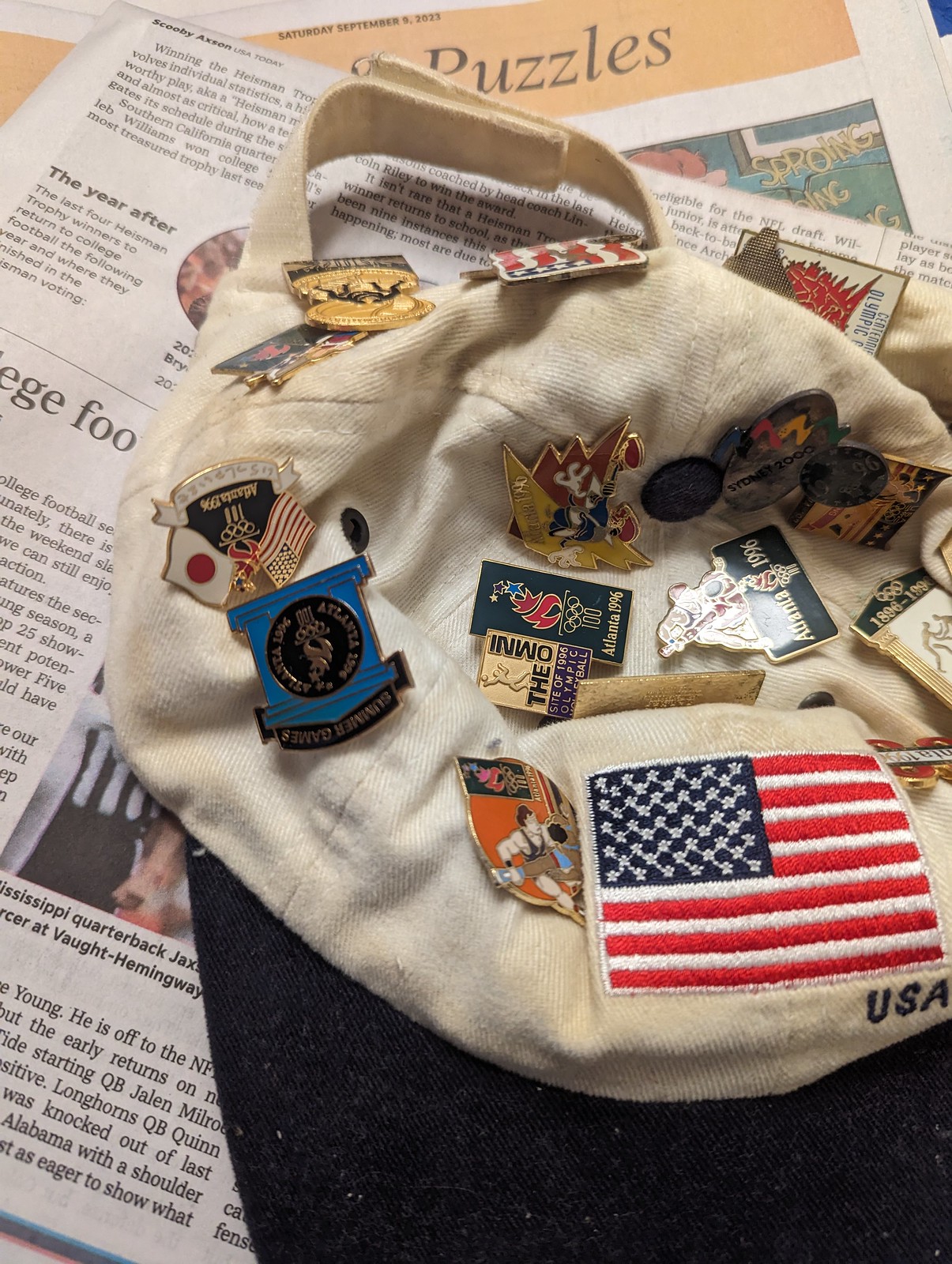The image presents a light beige baseball cap adorned with a variety of pins, prominently featuring a patch of the American flag with "USA" inscribed below it. The front of the hat is black or navy blue in color and hosts a collection of pins primarily from different Olympic events. Notable pins include those from the 1996 Atlanta Olympics, the 2000 Sydney Olympics, and the Olympics in Japan. Among the pins are depictions of the Olympic torch, wrestling, and multiple US flag designs. The hat is resting on a stack of newspapers, adding a contextual background to the photograph.